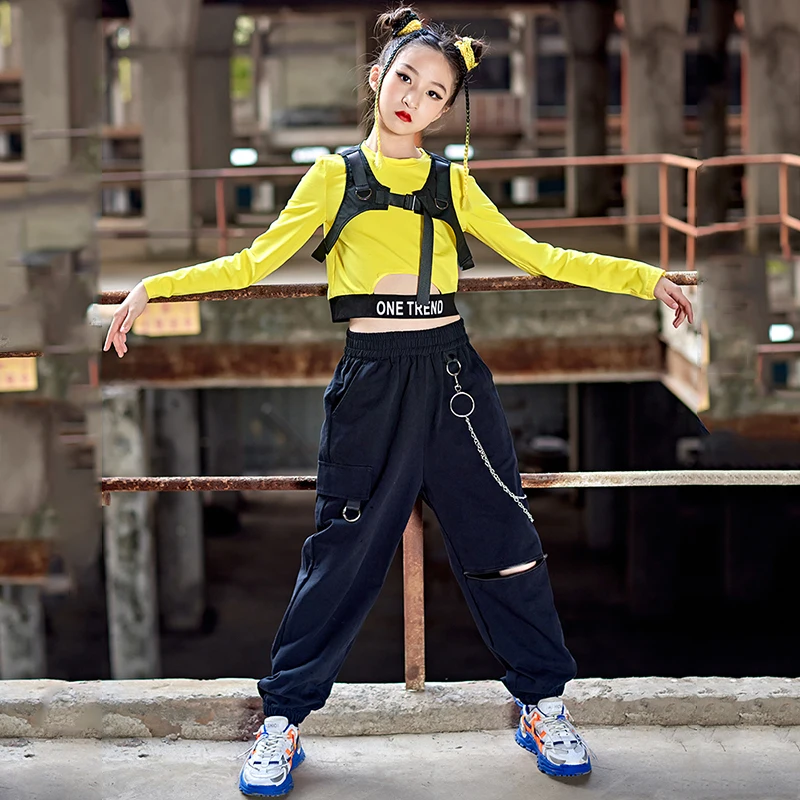The photograph features a young, slender woman standing in an industrial setting, potentially an old warehouse characterized by cement structures. She is posed against a rusted steel railing, resting her arms on it with her back to the metal. Her dark hair is styled into two pigtails, adorned with yellow hair ties, and extends downward in braids that frame her face tilted to the side.

The woman is dressed in a trendy, hip-hop-inspired outfit consisting of a yellow long-sleeve t-shirt partially covered by a black harness. The harness has a band at the bottom emblazoned with the text "One Trend." Her midriff is slightly visible between the shirt and a pair of blue stretchy pants. The pants, which feature a zipper over the left knee and multiple pockets, are accompanied by a chain hanging from the side. She completes her look with white and blue sneakers. The background is blurred, drawing focus to her stern yet stylish demeanor as she stands prominently in the center of the frame.